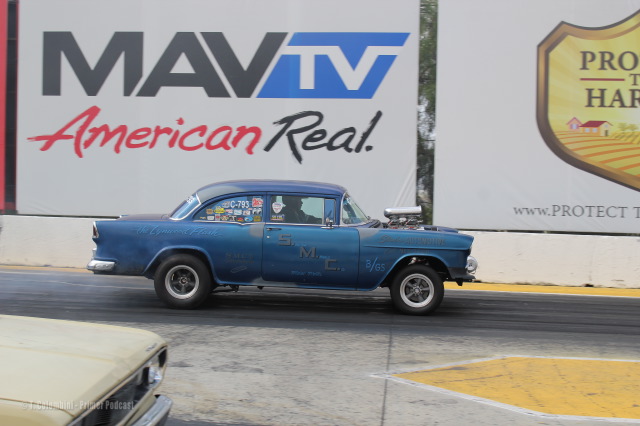The image depicts a vintage royal blue 1955 Chevy Bel Air, prominently featured with a chrome blower emerging from an open hood. The car is adorned with numerous stickers on the back window and along the passenger door, which also bears the text "SMC" in diagonal lettering. Its sleek two-door coupe design is captured in detail, showing well-maintained silver and gray rims. The scene takes place at a drag strip, indicated by the yellow and white road markings and the presence of another car's hood in the bottom left corner. A driver, visible with a helmet, sits ready inside the blue vehicle. In the backdrop, a sign reads "MAV TV American Real," and another billboard displays "www.protect" within a yellow badge, all set against a white wall highway barrier. The entire setup suggests that the car is either poised for a race or has just completed one, showcasing its pristine condition and the care it has received over the years.